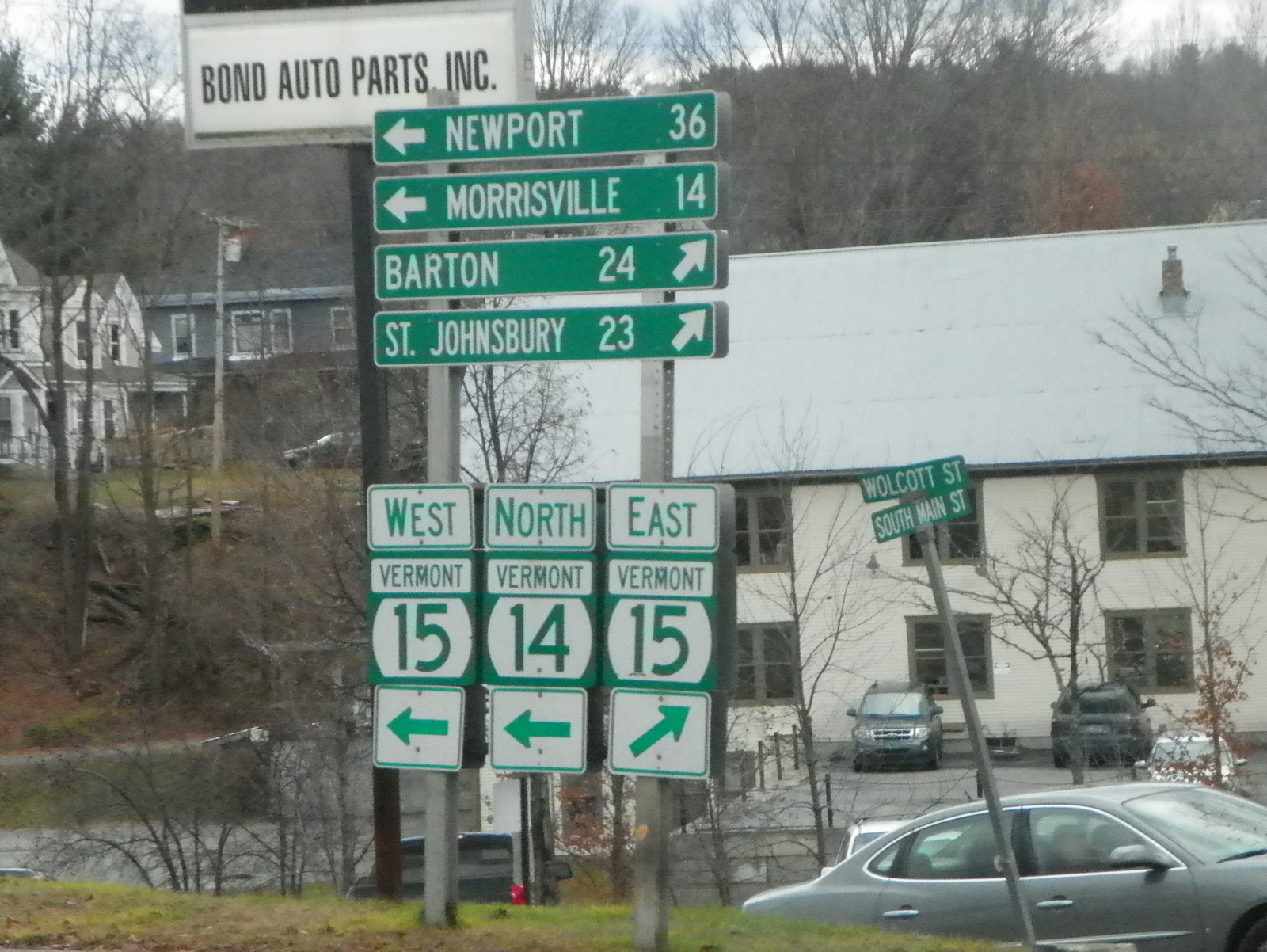In this image, a series of highway signs provide directions to motorists. An off-white building with a slightly lighter colored roof, topped with a small chimney, serves as the primary backdrop. This building features several gray windows and is adjacent to a small parking lot containing a few gray and silver cars. A prominent white sign with black lettering reading "Bond Auto Parts Inc." is mounted on a tall black post. The surrounding landscape includes leafless trees, indicating a season of dormancy. 

On the right side of the image, a silver post displays two green signs with white lettering, marking Walcott Street and South Main Street. At the forefront, multiple green highway signs deliver navigational information: one directs to Newport, 36 miles to the left, another points to Morrisville, 14 miles to the left, Barton, 24 miles with a diagonal upper-right arrow, and St. Johnsbury, 23 miles with an upper-right arrow. Additionally, signs indicate routes to West Vermont (15 miles to the left), North Vermont (14 miles to the left), and East Vermont (15 miles with an upper-right arrow).